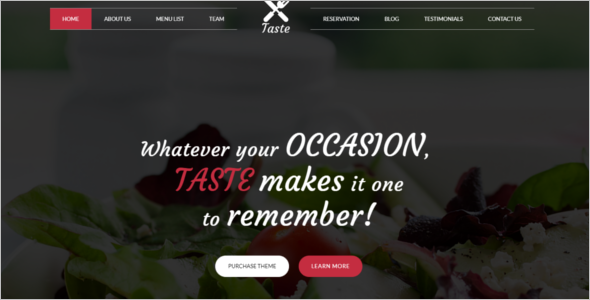The image depicts the homepage of a restaurant-themed website. The header features several navigational tabs including "About Us," "Menu List," "Plan," "Reservation," "Blog," "Testimonials," and "Contact Us." Dominating the top section is a distinctive logo consisting of a fork and knife crossed in an 'X' shape with the word "Taste" written beneath it.

The background of the webpage is a dark hue, partly obscured, but appears to feature an image of a salad in a white bowl. Overlaid on this background image is a bold text caption which reads, "WHATEVER YOUR OCCASION, TASTE MAKES IT ONE TO REMEMBER!" The phrase "TASTE" is highlighted in red, emphasizing the brand name.

Below the caption, there are two prominent buttons: a white "Purchase This Theme" button and a red "Learn More" button with white text. These call-to-action buttons suggest that, alongside its restaurant focus, the site may also offer website themes for purchase. However, the presence of reservation features and other restaurant-related sections confirms its primary function as a restaurant website.